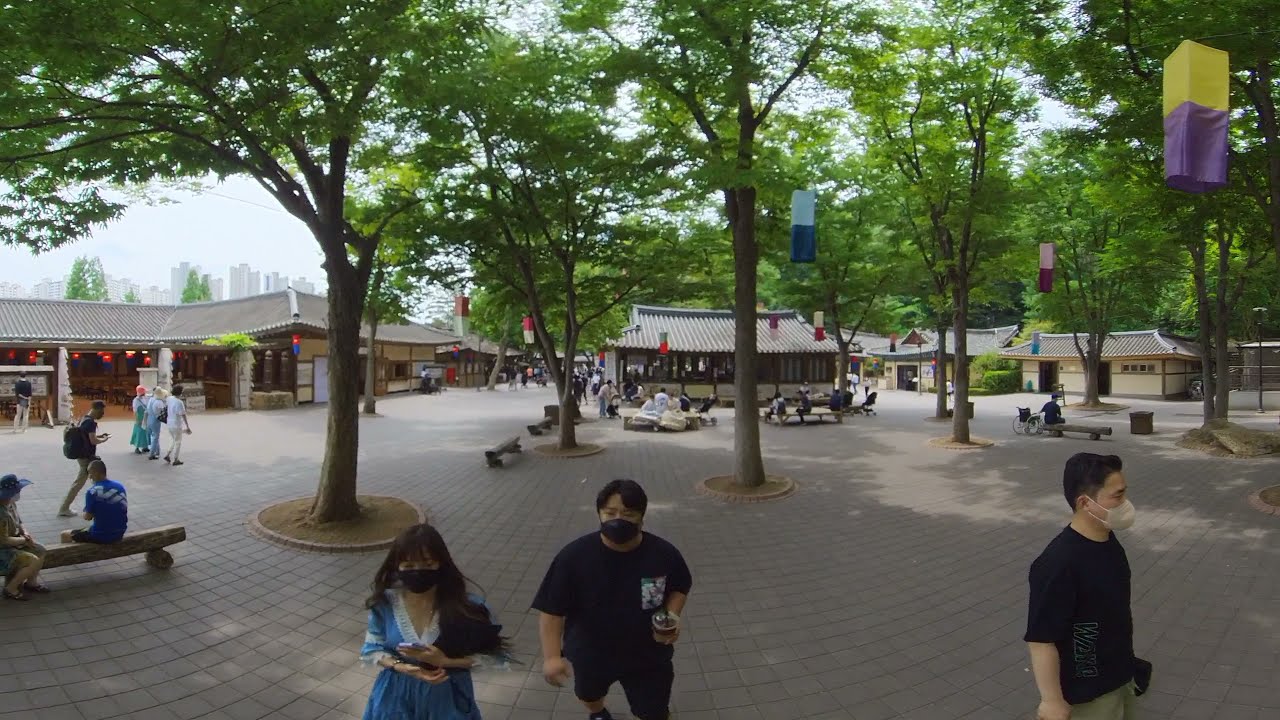This outdoor photograph, likely taken in an Asian country such as Japan based on the architectural style, captures a bustling park or plaza scene. The area is adorned with numerous one-story buildings featuring distinctive pagoda-shaped, terracotta or gray roofs. The foreground showcases two men wearing black shirts and face masks, and a woman in a blue dress, also masked, holding a cell phone. To the woman's left, two more individuals sit on a log bench while other people can be seen walking away in the background.

The scene is shaded by numerous green trees, each surrounded by cobblestone pathways and bordered by small concrete edges and dirt. Some trees have decorative, cloth-like banners or hanging lanterns adding a festive touch. The ground is largely paved, providing space for scattered log benches. The image also reveals open buildings with porch areas, possibly shops, where people are seated. In the far background, a city skyline with tall buildings can be discerned under a gray sky, completing this vivid depiction of a lively park setting.